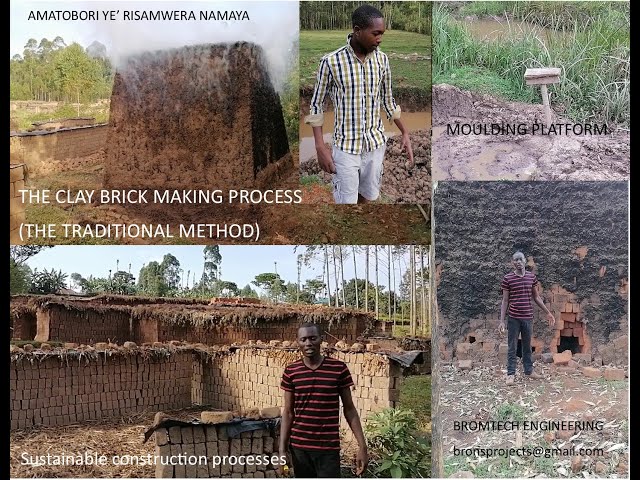The composite image, consisting of four distinct sub-images laid out as if from a magazine page, vividly captures the traditional clay brick-making process, likely set in an arid, outdoor environment reminiscent of Africa. The main image, occupying the top left, shows a smoldering clay mound used as a kiln, and is labeled in black font with "Amatobori" and in white font "The Clay Brick Making Process (The Traditional Method)." Adjacent to this, on the top right, a smaller square image features a text "Molding Platform" next to an image of a wooden pole protruding from a muddy area, signifying the initial clay shaping stage.

Below the main image on the left, another photo showcases a man in a black and orange striped shirt with black pants. He stands in front of stacks of bricks and a rustic hut, representing a key player in this sustainable construction process. The caption here, in white font, reads "Sustainable Construction Process."

To the right of this, the same man is again featured in a rectangular image, seemingly discussing the brick-making intricacies. This section is captioned "Brome Tech Engineering," with an email contact "prospects@gmail.com."

The images collectively depict the entire brick-making sequence—from extracting and molding the clay, steaming out moisture, to drying the finished bricks against a dry, desert-like backdrop with forested areas visible in the background.